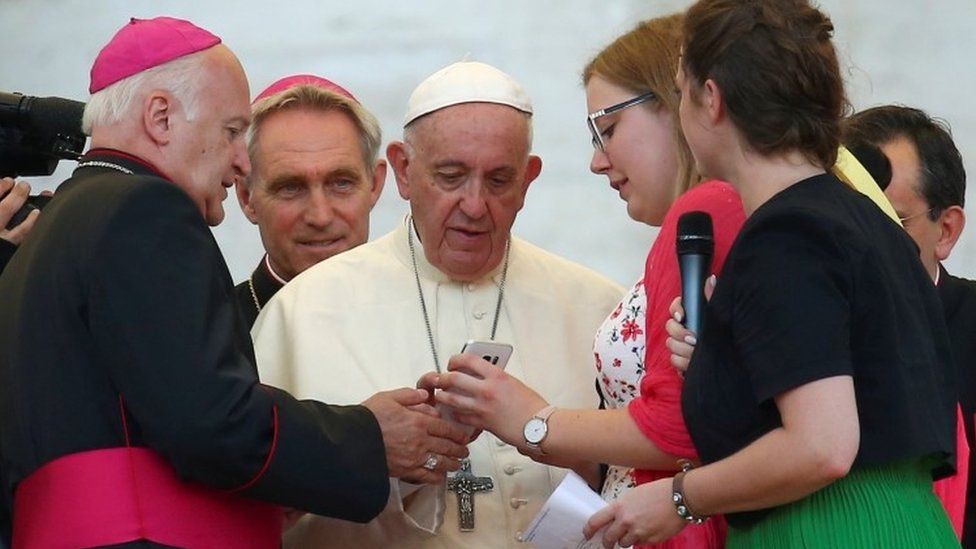In this captivating image, the Pope, dressed in his traditional white attire and adorned with a prominent silver cross around his neck, stands at the center of a gathering during an outdoor speaking event. He is encircled by a diverse group of individuals, including two cardinals on his right and two women on his left. The cardinals are attired in black gowns with red sashes and red caps. One of the women closest to the Pope is holding a microphone, while the other, positioned slightly behind, is presenting something to the Pope on a small white smartphone. The Pope, deeply focused, is holding the phone with careful assistance from the cardinal on his left, who ensures that the phone is securely held. The second cardinal in the background observes the scene attentively. To the far right, a camera partially enters the frame, capturing the moment. The women are dressed in vibrant colors, including green and a flower-patterned dress. The scene is lively, with everyone appearing respectful and engaged as they surround the pontiff amid a backdrop that suggests they are outside, filled with a bright white ambiance.